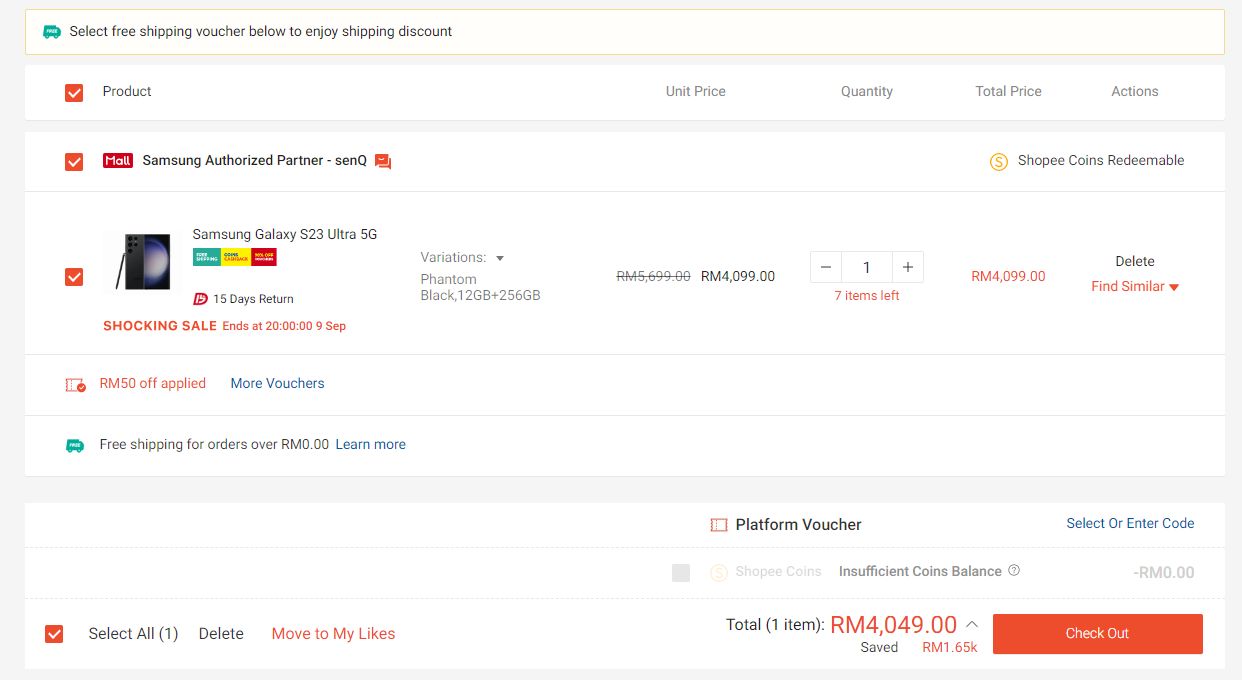At the top of the image, a tan rectangle with a yellow border features an icon of a green truck alongside text that reads, "Select free shipping voucher below to enjoy shipping discount." Below this, there is a structured table with columns labeled: Product, Unit Price, Quantity, Total Price, and Actions.

To the left of the 'Product' label, a red checkmark enables the selection of all items in the basket. The basket contains two items, both marked with red checkmarks indicating their selection.

1. **Samsung Authorized Partner – Send Queue**: 
   - Next to the unit price, a yellow circular icon with a dollar sign indicates that Shopee coins are redeemable.

2. **Phantom Galaxy S23 Ultra 5G**:
   - Accompanied by a picture of the box, and a small, unreadable text box in green, yellow, and red colors.
   - Text below the product name states, "15 days return."
   - An alert below this states, "Shocking sale ends at 20:00, September 9th."
   - To the right of the product name, the text "Variations" is followed by the specification "Phantom Black, 12GB + 256GB."
   - The unit price is listed as RM4099.00.
   - Quantity is set to one, with plus and minus buttons for adjustment. A note underneath indicates "7 items left."
   - The total price mirrors the unit price at RM4099.00.
   - Next to the total price, options include a delete button and a "find similar" pop-up.

Below this table, text indicates an applied voucher offering RM50 off, along with options to apply more vouchers and details about free shipping for orders over RM0.00.

At the bottom of the list, a white box labeled "Platform Voucher" allows users to select or enter a code. Below this, buttons are available to "select all," "delete," or "move to my likes." The summary section indicates a total of one item, with the final price listed as RM4049.00, showing a saving of RM1650.00 (RM1.65K). Lastly, a prominent checkout button is displayed for finalizing the purchase.